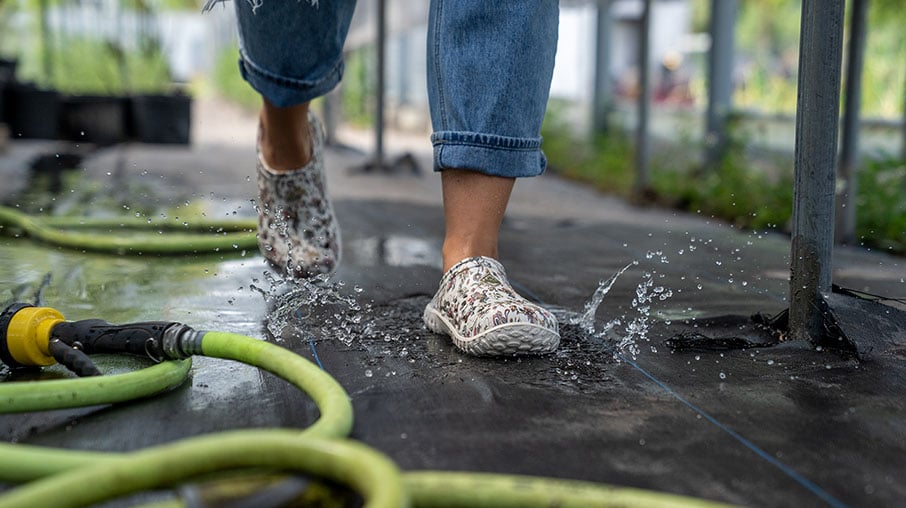This photograph captures a ground-level view of a person walking through a greenhouse. The focal point is the individual’s feet and legs, clad in cuffed blue jeans that end high above the ankle. They are wearing slip-on shoes with a white base and a printed design on the upper portion. The person is splashing through puddles on the greenhouse floor, which is covered in black weed guard material. In the lower left-hand corner, a light green garden hose with a yellow and black spray nozzle coils on the ground. Blurred potted plants and greenery populate the upper sections of the photo, adding a vibrant backdrop to the earthy and serene scene.